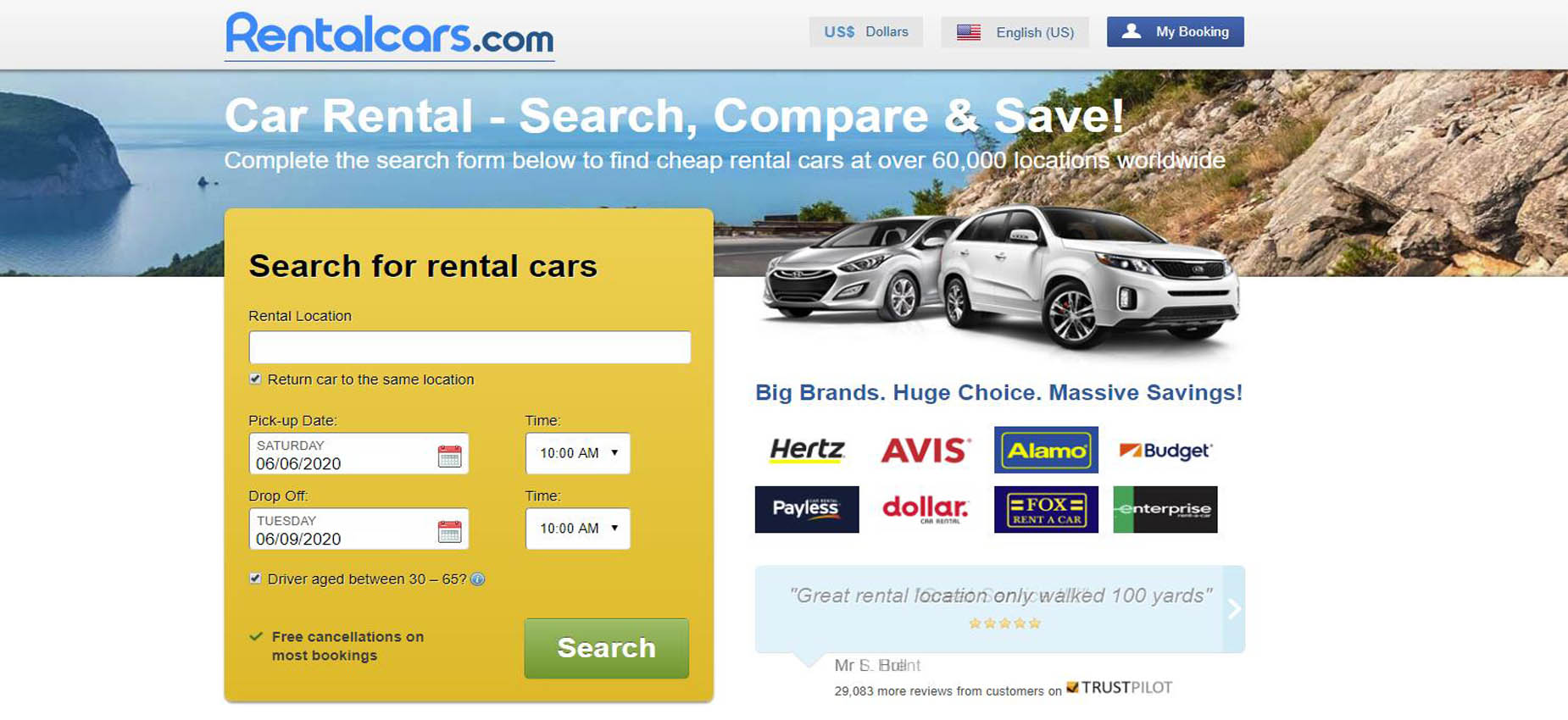The webpage for Rentalcars.com features a clean, user-friendly interface for booking rental vehicles. At the top, there is a gray navigation bar with the "Rentalcars.com" logo, where "Rentalcars" is in blue text and ".com" is in black. On the right side, the user can select the currency (USD) and the language (English), marked by an American flag icon. Additionally, there's an option to view the user's itinerary under a profile icon.

Below the navigation bar, a vibrant header image spans the width of the page, depicting a scenic coastal highway flanked by mountains and water. Superimposed on this image is the website's slogan in bold white text: "Car Rental - Search, Compare, and Save!"

Following this, white text invites users to "Complete the search form below to find cheap rental cars at over 60,000 locations worldwide." 

Underneath, a prominent yellow box encourages users to "Search for Rental Cars" in black text. The search form itself includes fields for location, pick-up date and time, and drop-off date and time. At the bottom of the form is a green search button labeled "Search" in white text. Adjacent to this, two car icons display branded logos, showcasing options available for rental.